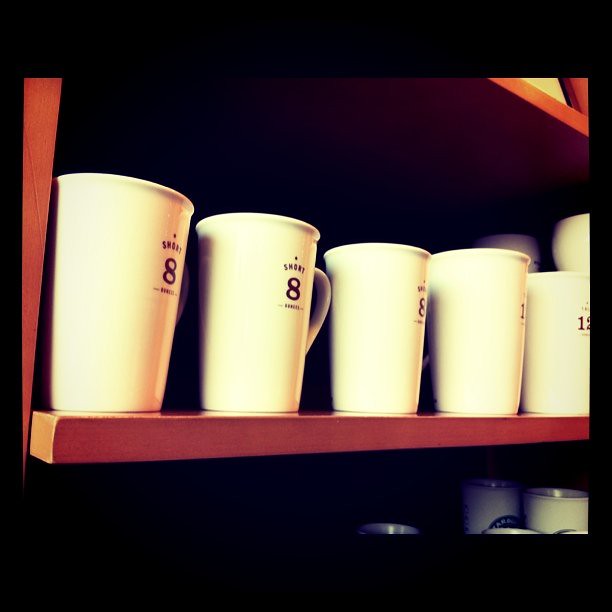The photograph displays a square, color image of a three-tier wooden shelf with a reddish finish. The primary focus is on the middle shelf, which prominently features a neat lineup of ten tall, creamy yellow cups, each adorned with a logo that reads "Short 8," accompanied by an illegible word beneath. These cups resemble coffee mugs, each equipped with a single, slim handle. The material of the cups is indeterminate, suggesting they could be made of plastic or porcelain. Below this shelf, just the tops of various other objects, possibly beverage cans or metal tumblers, are partially visible. The shelf’s left support, matching the reddish wood finish, is partially in view. In the upper right corner of the image, a small triangle of yellow peeks out beyond the shelf’s edge, adding a touch of intrigue to the composition.